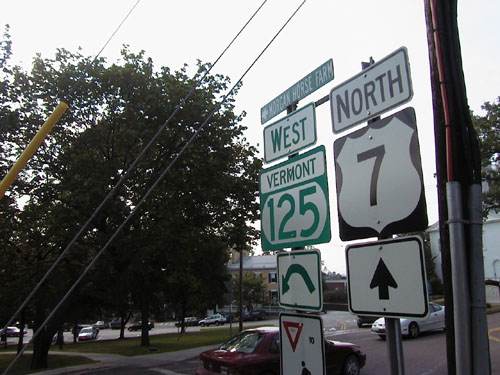This rectangular photograph, oriented with the longer sides extending from left to right, captures a series of road signs against a backdrop of trees and parked cars. In the foreground, two poles are visible among the signs. The pole on the far right is partially gray and red, feeding into a base brown support, and appears to carry electrical wires.

The first sign from the top left reads "North" above a black and white highway shield marked with the number "7" and an upward-pointing arrow. Adjacent to it, the other pole hosts multiple signs: at the top, a green street sign with white text referring to "[something] Farm." Below it, a larger sign displays "West" in green text on a white background with a green border, followed by the words "Vermont" in white on green and the number "125" below. Underneath these, a green arrow indicative of a U-turn appears. At the very bottom of this pole, a white sign features a red-bordered yield triangle with a black pedestrian symbol inside.

In the background, we see a couple of parked cars, one red and one white, surrounded by tall trees. Supporting cables arc from the pole at the far right into the upper middle of the composition, providing structural integrity. The overall scene includes a hazy sky above a visually busy roadside setup.